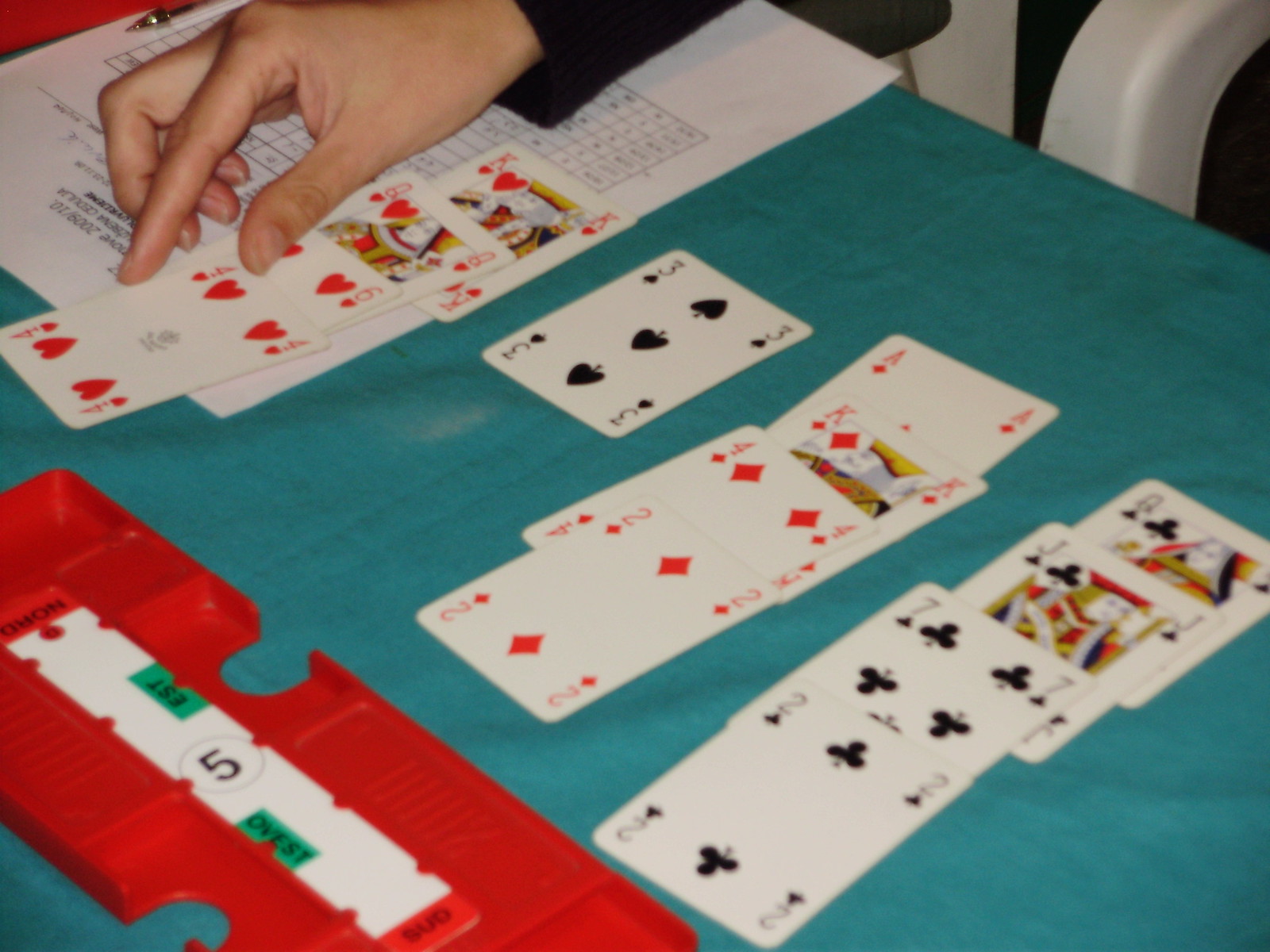This image captures a game of solitaire in progress, played on an emerald green cloth spread over a table. At the center of the table, a three of spades stands apart from a scattered set of cards, which includes an ace, king, four of diamonds, and two of diamonds. Towards the bottom right, a tightly stacked pile reveals a sequence featuring the two of clubs, seven of clubs, jack of clubs, and queen of clubs. A hand, clad in a black sleeve, is seen interacting with the cards, presumably contemplating the next move. In the upper right corner, a chair with a white armrest and a white wall is partially visible. The top left of the image presents a hint of red from an unidentified source. Nearby, a white piece of paper with black printing lays beside a silver pen. Additionally, in the bottom left corner, a red tray holds a card or sheet adorned with a white background, red spots, green sections, and red dots.